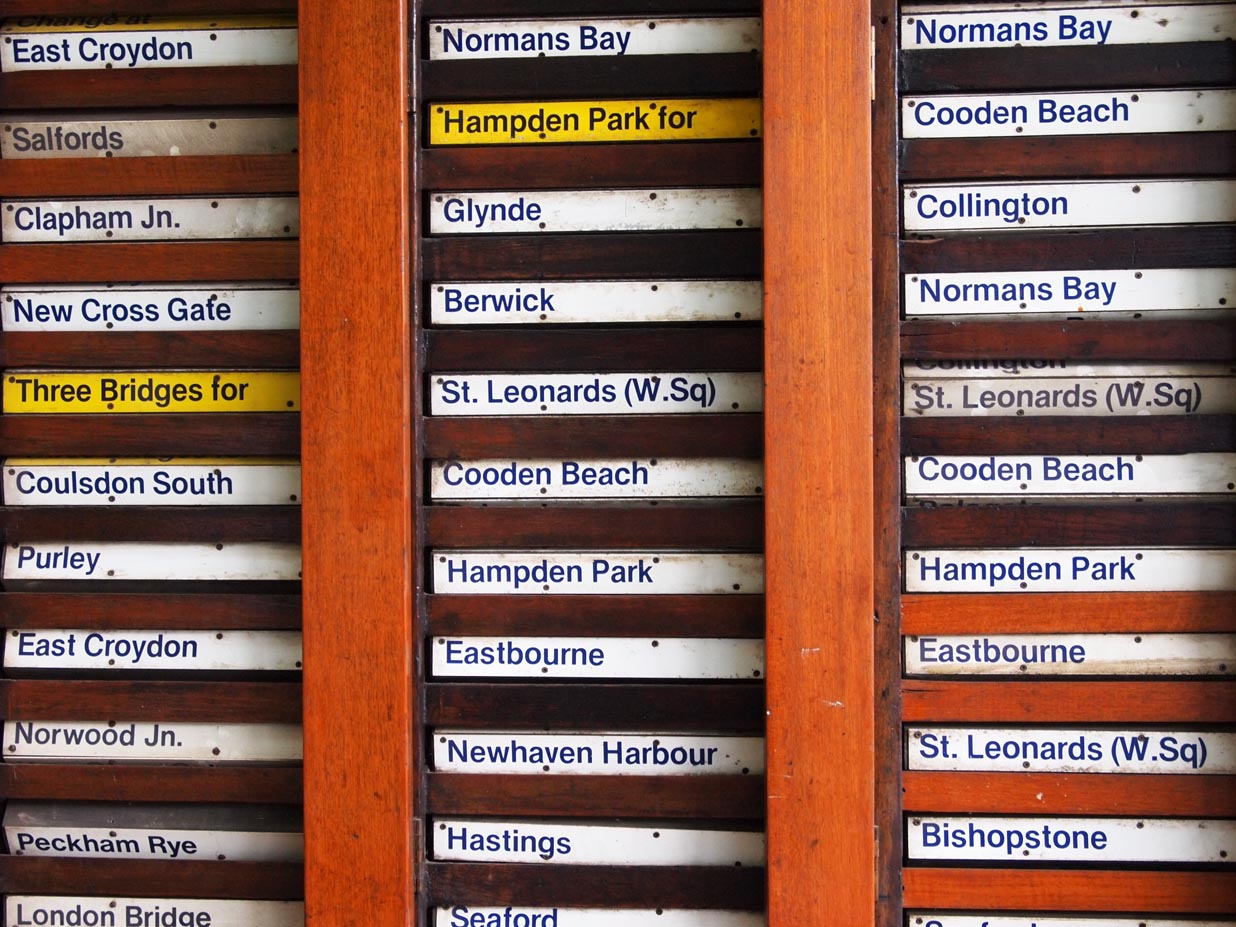This image showcases a detailed destination grid made of wood, featuring three vertically separated columns of destination names. The vertical slats separating each row and column are made of wood, creating a structured and orderly layout. Each destination is listed on a placard, with a mix of backgrounds and text colors: blue lettering on a white background, black lettering on a white background, and black lettering on a distinct yellow background.

In the leftmost column, the destinations listed from top to bottom are: East Croydon, Salford’s, Clapham Junction (JN), New Cross Gate, Three Bridges 4 (with a yellow background), Coulson South, Purley, East Croydon, Norwood Junction (JN), Peckham Rye, and London Bridge.

The central column features the following destinations from top to bottom: Norman’s Bay, Hampton Park 4 (with a yellow background), Glynd, Berwick, St. Leonard’s West Square, Eastbourne, New Haven Harbor, Hastings, and Seaford.

Finally, the rightmost column presents these places from top to bottom: Norman’s Bay, Coudon Beach, Collington, Norman’s Bay, St. Leonard’s West Square, Coudon Beach, Hampton Park, Eastbourne, St. Leonard’s West Square, Bishopstone, with the bottom-most entry being cut off and unreadable.

The destinations appear to be listed on what looks like cassette tape-like placards, giving an impression of an organized system, likely for tracking or indicating train destinations.